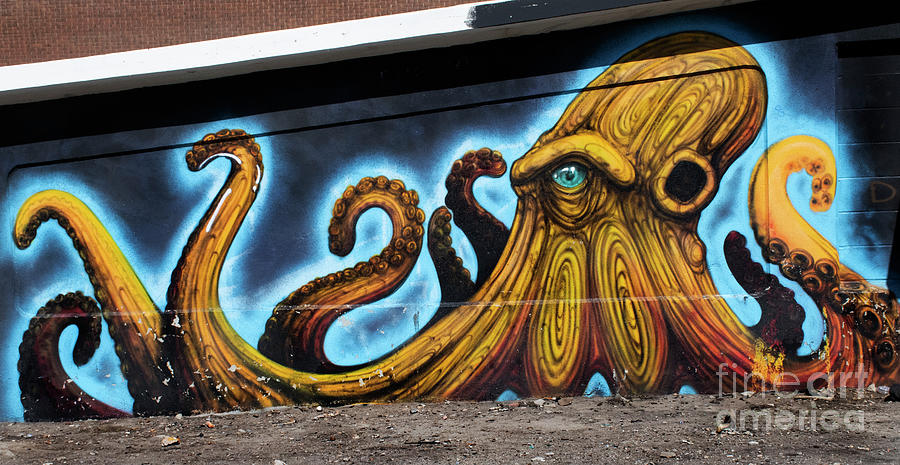This image captures a detailed and vibrant graffiti mural of an octopus on a weathered brick wall. The scene is set outdoors with the brick building slightly visible towards the top left, suggesting the artwork adorns the side of a building. The ground in front of the wall is dirty, littered with debris and chunks of rock, adding to the neglected atmosphere. The mural itself is striking, featuring a yellow and brown octopus with one prominent blue eye. There's an enigmatic hole or opening to the right of the eye, the purpose of which is unclear. The octopus is set against a blue background with varying shades that darken almost to black around the edges, and the top border of the wall is half black and half white. The octopus is depicted with three tentacles reaching towards the left, three stretching mid-frame, and two trailing off towards the right edge. A watermark from "Fine Art America" is visible in the bottom right corner, underscoring the mural's aesthetic value.